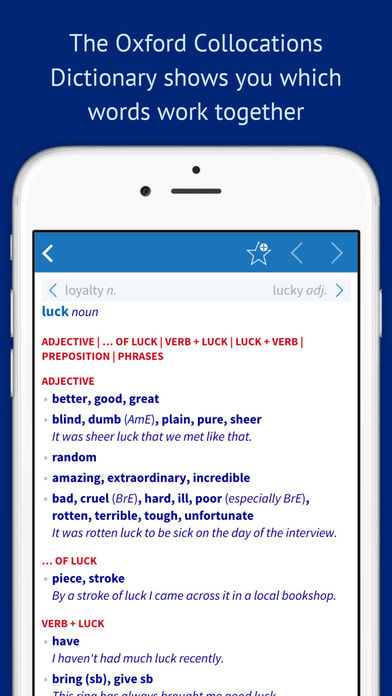The image features a blue background with a header that reads, "The Oxford Co-Location Dictionary shows you which words work together." Below this header, there is an illustration of a white smartphone. The smartphone's screen displays a blue border at the top with icons including a left-facing arrow (<) on the left, a star in the center, and a greater than symbol (>) on the right. Below these icons, the main content on the smartphone screen is shown, detailing lexical collocations for the word "luck." The text on the screen breaks down the use of "luck" as both a noun and an adjective (A-D-J), with examples such as "adjective of luck," "verb plus luck," and "prepositional phrases." Examples provided include various adjectives that can be used with "luck," such as "better," "good," "great," "blind," "dumb," "plain," "pure," "sheer," and illustrate usage with sentences like "It was sheer luck that we met like that." Negative adjectives include "bad," "cruel," "hard," "ill," "poor," "rotten," "terrible," "tough," "unfortunate," with a usage example: "It was rotten luck to be sick on the day of the interview..." Finally, the screen presents phrases like "stroke of luck," used in the sentence "By a stroke of luck I came across it in a local bookshop."